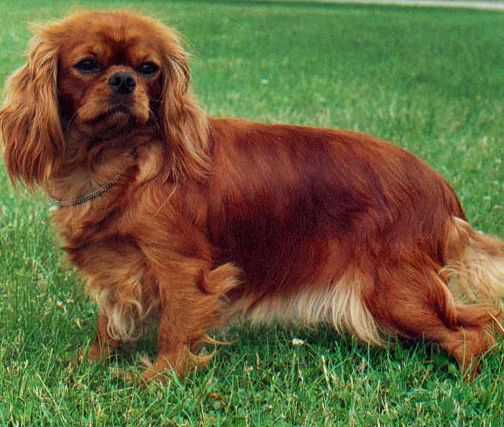This captivating photo features a small, fluffy puppy with a striking golden brown coat that leans towards a reddish hue. The puppy is standing in the center of a lush, green grassy area, speckled with small white flowers and occasional weeds. The fur on its ears is long and rich in texture, complementing its dark, chocolate-brown eyes and a cute, smooshed nose. The dog's head is positioned towards the top left of the image, gazing directly at the camera, while its body faces left, showcasing its silky, lighter-colored fur hanging from its belly. The reddish tint in its back fur transitions to white or blonde underneath, creating a beautiful contrast. The puppy's tail, bushy and of a lighter tan shade, is slightly cropped off on the right side of the frame. A thin silver chain collar adorns its neck, underscoring its endearing charm. The background of verdant grass with patches of brown further highlights the puppy's colorful fur.